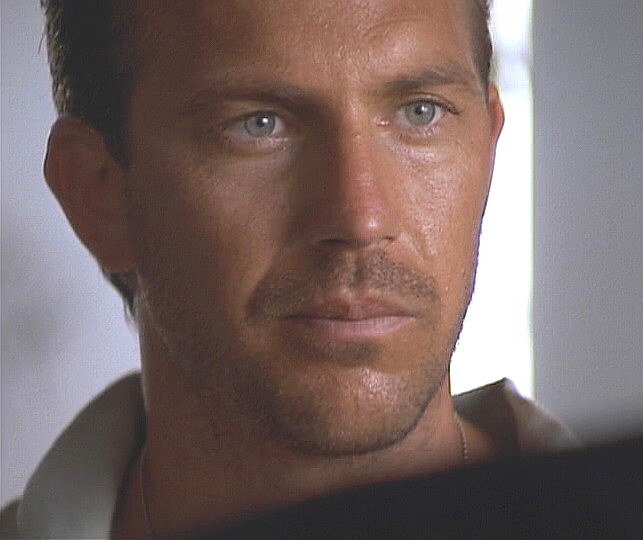The image captures a younger Kevin Costner, likely during one of his 1980s films. He is wearing a cream or white collared shirt complemented by a small beaded silver necklace. Costner has piercing blue eyes and a neatly trimmed beard and mustache, which give him a rugged yet polished look. His hairstyle is short but not a buzz cut. The background is blurred, showcasing the edge of a wall and hints of something blue, drawing focus solely to Costner. The bright lighting behind him and the indistinct details suggest this is a movie scene from one of his roles, possibly from films such as "Revenge" (1989) or "No Way Out" (1987). A black spot, resembling a 90-degree triangle, is visible in the bottom right corner, adding an element of intrigue to the composition.